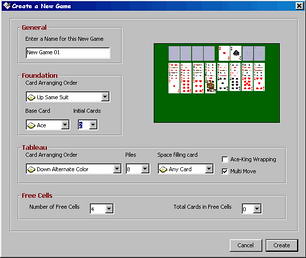This image depicts a computer screen displaying a program interface for creating a new solitaire game. The top section features a blue bar with the text "Create a New Game" on the left. On the right side of the screen, a Solitaire card game is showcased on a green backdrop. The game features several vertical piles of face-up cards beneath a horizontal row comprising mostly face-down cards, with two cards face-up.

On the upper left section of the screen, maroon text reads "General," followed by black text stating "Entry" and "Name for the new game," which is displayed above a white text box labeled "New Game 01." Directly below this, maroon text denotes "Foundation," with black text indicating "Card Arranging Order." The area includes additional text that is too small to decipher.

Towards the bottom, another section titled "Tableau" involves instructions for card arranging order. Further below, it details "Free Cells," specifying the number of free cells and the total cards in the free cells. At the bottom-right corner, two buttons labeled "Cancel" and "Create" are visible. The background color of the screen is gray, providing a neutral backdrop to the interface elements.